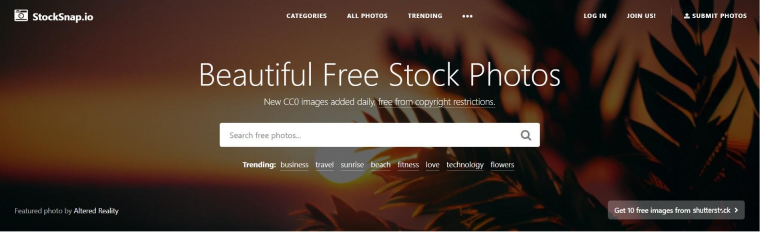The image is a screenshot of the homepage of a website named "Stocksnap.io." At the top left corner of the page, the website name "stocksnap.io" is prominently displayed. Centrally located near the top is a navigation menu offering different categories, including "Categories," "All Photos," and "Trending," followed by an icon of three dots indicating additional options. On the right side of this top bar, there are links for "Log In," "Join Us," and "Submit Photos." 

Below this upper navigation bar, a large title reads "Beautiful Free Stock Photos," with a subheading underneath stating "New CCO images added daily, free from copyright restrictions." Positioned directly below this introductory text is a large search bar with the placeholder text "Search for free photos," inviting users to search the website's stock photo collection. The overall design is clean and user-friendly, emphasizing the availability and accessibility of high-quality, copyright-free images.